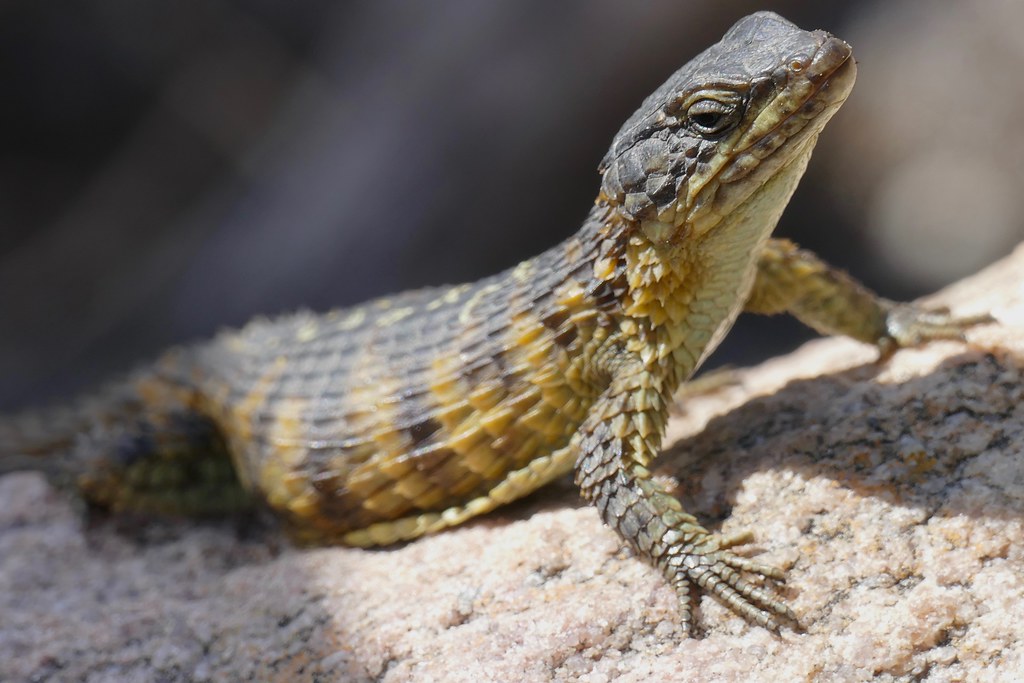The image captures a close-up shot of a lizard basking in the bright outdoor daylight. The background is intentionally blurred to emphasize the lizard, which stands out clearly on a rough, gravel-like surface. This green lizard, covered in sharp, scaly textures, exhibits a spectrum of colors ranging from light green to dark green with hints of brown. It has its little hands prominently displayed on the right side of the image, and part of its tail is visible toward the left, though it is somewhat obscured. The natural lighting enhances the detail of its scaly surface, showing the lizard seemingly enjoying the sunny environment.